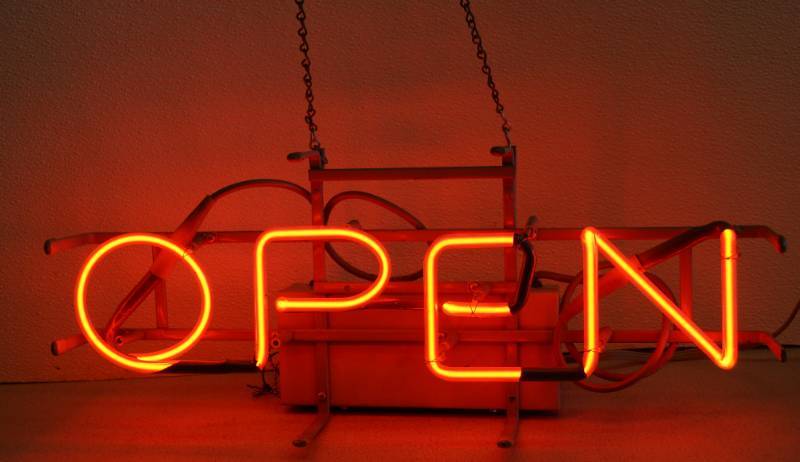This image features a close-up of an illuminated neon sign displaying the word "OPEN" in all capital letters. The sign emits a vibrant reddish-orange glow, with the intense center of each letter appearing yellow due to the brightness of the neon light. The background hosts a gradient of deep red to orange, fading into black towards the top, contrasting with the predominantly gray and slightly red-toned wall. This sign is suspended by metal chains, possibly giving the illusion of hanging or being part of a suspended storefront display. Additional metallic brackets are visible at the bottom of the frame, contributing to the industrial aesthetic. The surrounding environment is dark, but the neon light suffuses the space with a distinctive reddish hue. The sign is set against a backdrop that creates the impression of an undefined product or item, potentially interpreted as a trunk or chest, enhancing the mystery and allure of the scene.